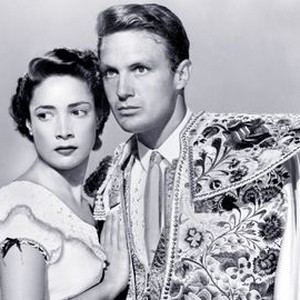This is a small, square black and white photograph likely from the 1960s, featuring a man and a woman standing closely together with their heads touching. The woman, positioned on the left, has short, dark hair slightly curled at the top and wears stud earrings along with a white dress that frills around the shoulders. She gazes sharply to her right, with a serious expression on her face. Her right hand rests gently on the man’s chest. The man, on the right, has short hair and also bears a serious expression as he looks to his left. He is dressed in a very ornate, intricately embroidered jacket adorned with floral patterns, and beneath it, he wears a white collared shirt and a tie. The background of the photograph is a solid, medium gray color.